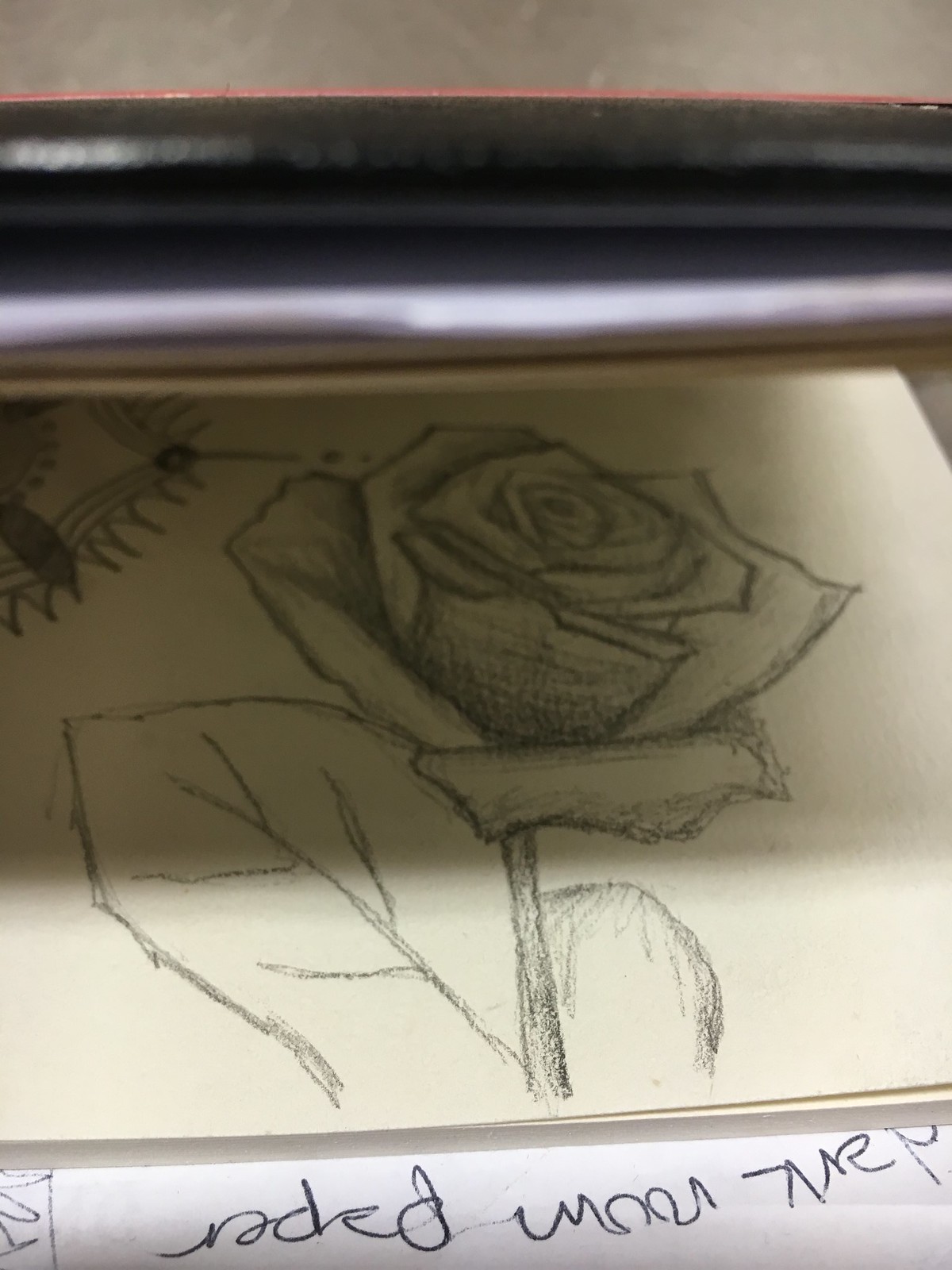This photograph captures a highly detailed pencil drawing of a rose, rendered in shades of gray and black on a cream-colored sheet of paper. The rose is intricately shaded, providing depth and a semblance of three-dimensionality, especially around the center of the bloom. A stem extends downward from the rose, with a less detailed leaf on the left and a partially visible leaf on the right. There is additional sketching in the upper left corner resembling either something like a postage stamp or an insect reaching for the flower. The drawing is viewed under a surface that casts a shadow across the top, blurring some details and making the lighting uneven. The image is set against a piece of white paper with barely legible, upside-down text that seems to read "Mark Now Paper." The drawing appears to occupy nearly half of the page, with faint elements suggesting it is part of a sketchbook or notebook, indicated by the visible edge of additional pages at the top.